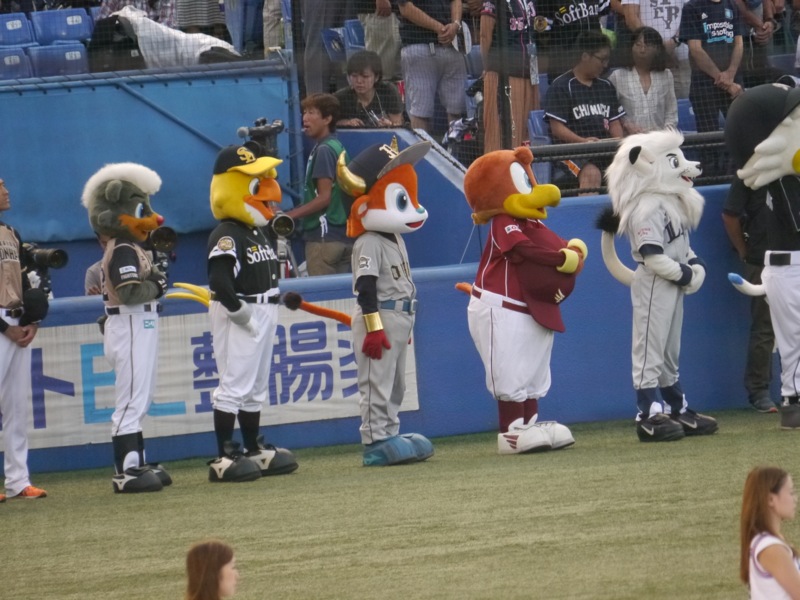This vibrant live color photograph captures a captivating scene at a professional baseball game during the daytime. In the foreground, seven mascots stand in a horizontal line on a meticulously maintained, light green field, seemingly participating in the National Anthem ceremony. The mascots, dressed in various colorful and oversized costumes, include characters such as a giant chipmunk, a rooster, a white lion, a squirrel, and a bird with a black hat. One notably dons a yellow chicken costume with the white text "Softbank" emblazoned on its chest.

Behind the mascots, baseball players are standing in respectful attention, some with their hands at their sides, likely paying homage to the anthem. A couple of mascots have even removed their hats, further indicating the ceremonial nature of the moment. The backdrop reveals vibrant stadium stands filled with spectators, with several individuals also standing, enhancing the sense of a shared patriotic or significant moment.

Adding to the dynamic atmosphere, a photographer clad in a green vest and blue shirt can be seen intently focusing his camera from behind a blue wall. A couple of cameras from the press box are also visible in the background, aiming to capture the essence of the event. The overall scene depicts a moment of unity and tradition, vividly showcasing the intersection of sport, entertainment, and patriotism.